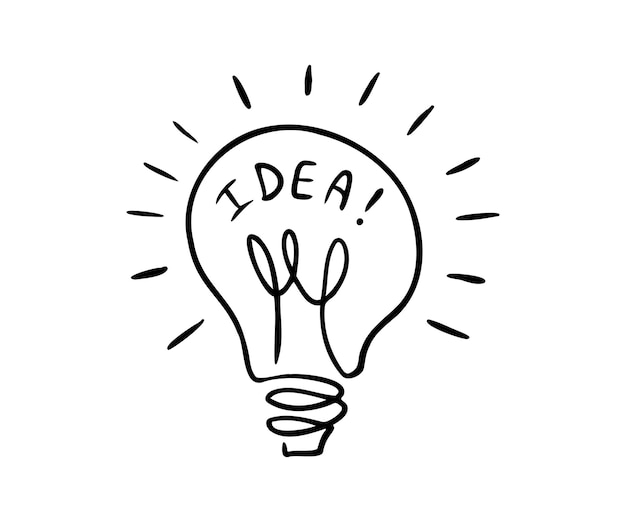The digital image is a simplistic, black-and-white line drawing of a light bulb. This basic illustration features clean, curved lines that outline the bulb, with two loops at the base representing the screw-in part. Inside the bulb, a squiggly filament adds detail, and surrounding the bulb are multiple dashes that convey it being lit. At the top inside the bulb, the word "IDEA" is prominently displayed in capital letters with an exclamation point. The overall composition is minimalist, with the black lines standing out starkly against a white background, emphasizing the concept of a bright idea with straightforward, unembellished artistry.